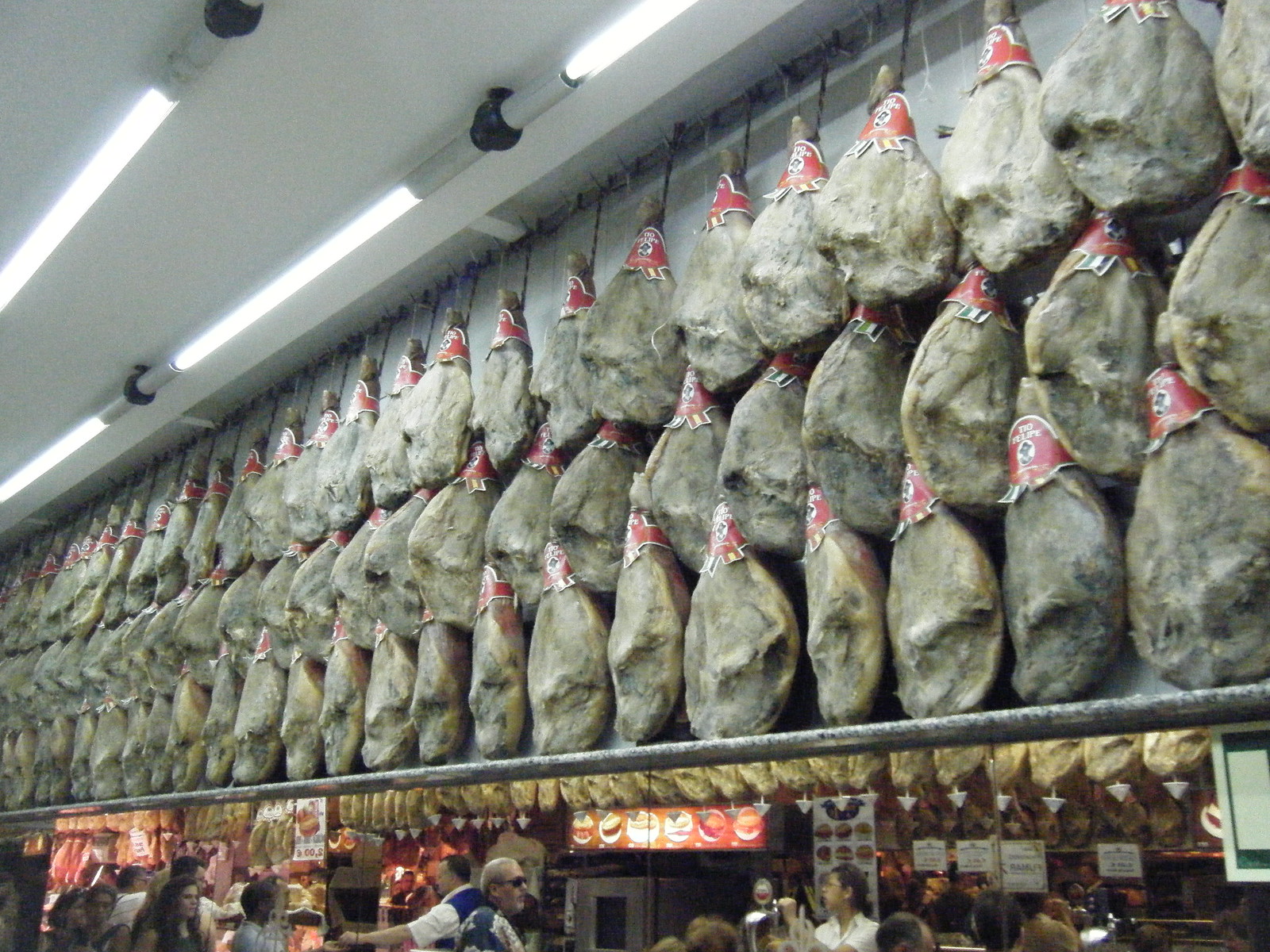The widescreen color photograph captures a bustling scene, tipped up slightly to reveal both the ceiling and the main focus: rows of suspended meat carcasses. The meats are prominently displayed across a long back wall, hanging in three horizontal rows from metal hooks attached to racking. Each carcass has a red label, possibly made of paper or cardboard, wrapped around its top. This visually striking setup suggests a setting in a meat market or butcher shop, potentially in an oriental or Far Eastern location.

Beneath the racks of meat, a portion of a restaurant or market environment is visible. Here, servers dressed in white tops are seen attending to patrons. The white ceiling features long fluorescent lights adding to the bustling atmosphere. While the activity below is partially obscured, glimpses of counters and food signage hint at a mixed-use space for both purchasing and consuming meat products. The detailed layering of the photograph, from the reflective surface of the meats to the activity beneath, offers a complex snapshot of a vibrant, multifaceted space.